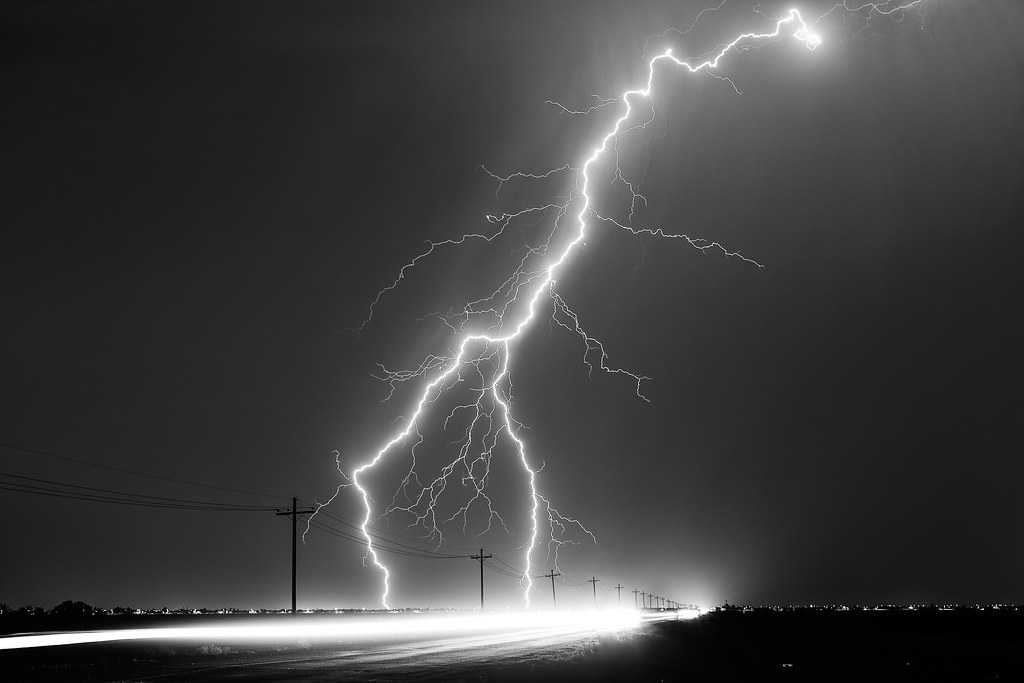This is a black and white photograph capturing an outdoor scene at night. The center of attention is a dramatic lightning bolt striking the ground, splitting into multiple streams about a hundred to a thousand feet above the ground. The main bolt illuminates the otherwise dark landscape, and two forks of lightning are particularly notable. The scene is set against a black sky and ground, with a road running through the middle of the image, flanked by electrical power lines. The road is animated by streaks of lights from passing cars, adding a dynamic element to the stillness of the night. The lightning appears to strike the left side of the road, creating a stark contrast against the gray-toned sky and the dark surroundings. The photograph, rectangular in shape and taken in landscape orientation, powerfully captures the raw energy and beauty of a lightning storm.